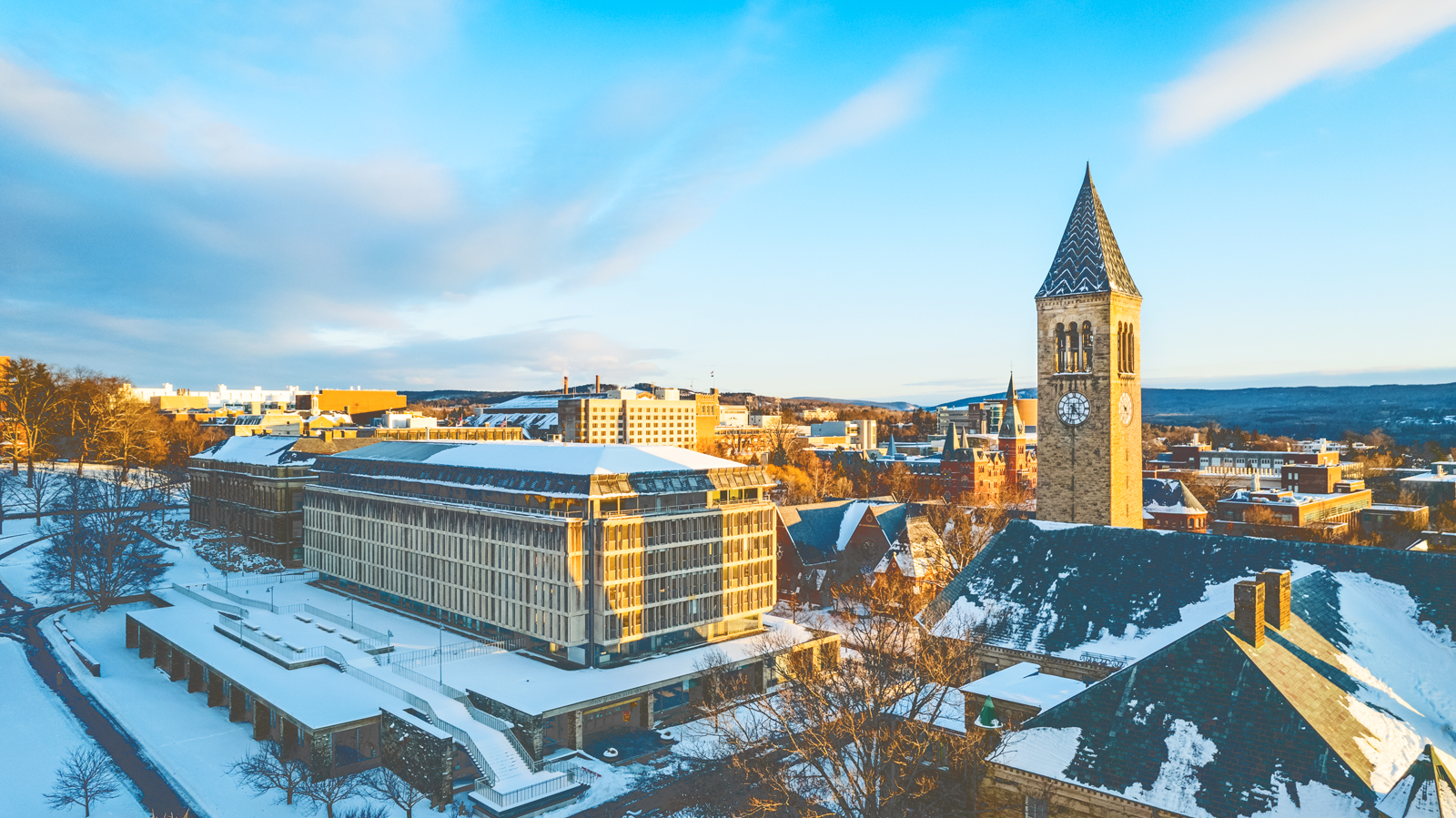The image captures a stunning, vintage postcard-like scene of a European town, taken from an aerial perspective, possibly by a low-flying airplane or drone. Dominating the right side of the frame is a snow-covered rooftop, behind which rises a tall clock tower with a pointed, slate roof and clocks on all its faces, resembling a historic steeple. To the left of the tower stands a distinctive, tan, four or five-story building, possibly a dormitory or library, characterized by its narrow windows. The town extends into the distance, featuring an array of modern and traditional tan buildings glistening under the sunlight, with snow dusting their roofs and the ground below. The vibrant blue sky is partly cloudy, adding a bright, clear backdrop to the serene winter scene. Bare brown trees punctuate the left side of the image, hinting at late autumn or early winter, while faint mountain peaks are visible in the far distance. The overall effect is a picturesque, nostalgic portrayal, reminiscent of colorful travel postcards from the 1970s or 80s.